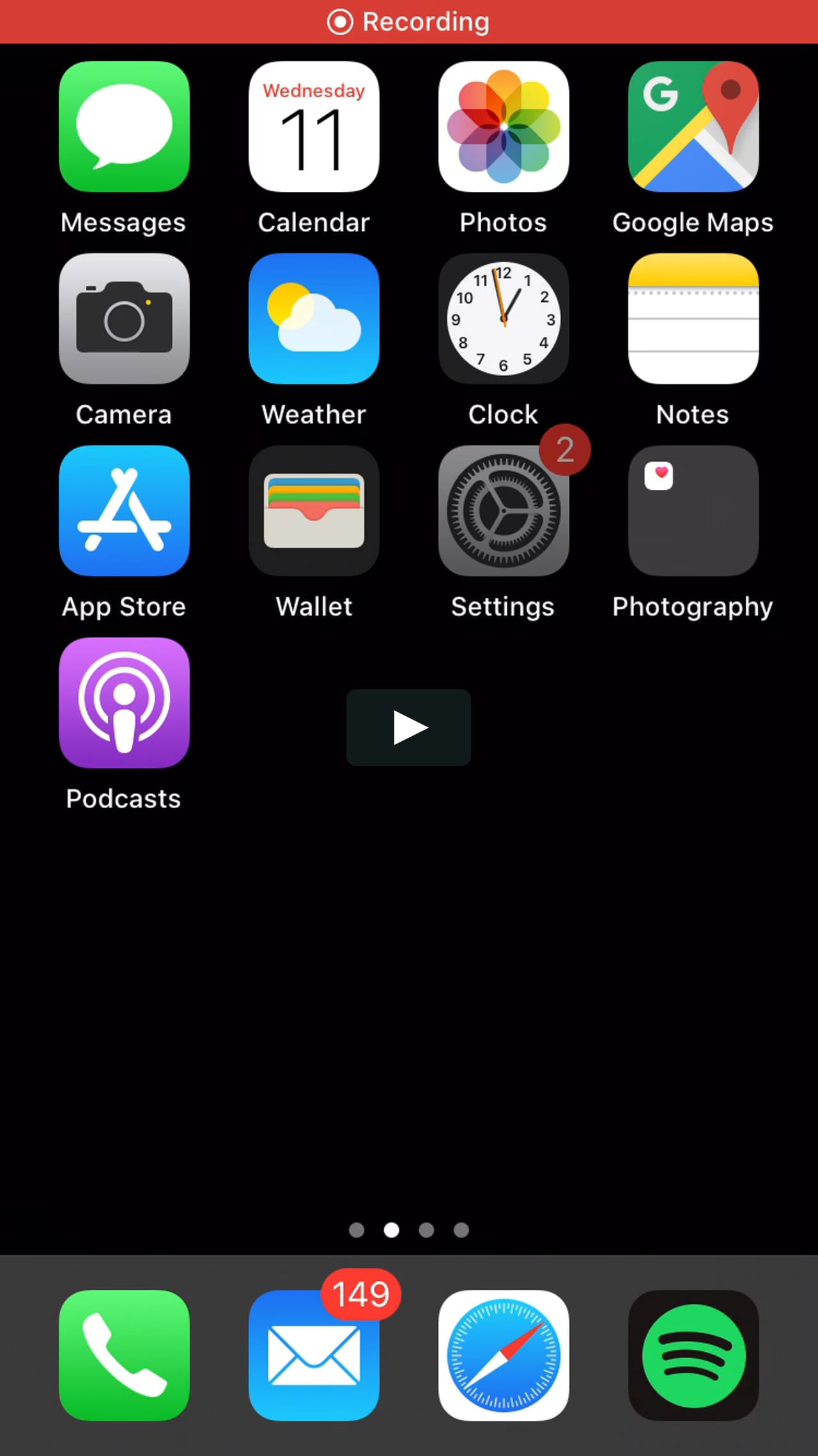The image portrays a mobile device's home screen set against a black background. At the top of the screen, a red strip featuring a white dot encircled in red and white, displays the text "Recording." Below this, several application icons are arranged in a grid format.

- **Messages**: Represented by a green box.
- **Calendar**: Shows the date as Wednesday the 11th.
- **Photos**: Icon is a multicolored star shape.
- **Google Maps**: Features a white "G" in the green corner, with additional yellow, blue, white, gray colors and a small red tag.
- **Camera**: Housed within a gray box.
- **Weather**: Shown in a blue box featuring a white cloud and a yellow sun.
- **Clock**: Standard clock icon.
- **Notes**: Depicted as a piece of white paper with a yellow top and blue lines.
- **App Store**: Displayed in a blue square with a white "A".
- **Wallet**: Icon is an image of a wallet.

Additional icons include:
- **Settings**: A gray square with a numeral "2" in a red circle indicating notifications.
- **Photography**: A black square with a white inner square containing a red heart.
- **Podcasts**: Illustrated in a purple square with a white person icon and circular markings.

Towards the bottom, there are four navigation dots, with the second one highlighted in white, indicating the current screen. Below this section, a gray bottom dock features:
- **Phone**: Green square icon.
- **Mail**: Blue square with an envelope, showing a red notification circle with "149".
- **An unidentified icon**: Resembling a thermometer in a blue circle with a white background.
- **Another unidentified icon**: A black square with a green circle within.